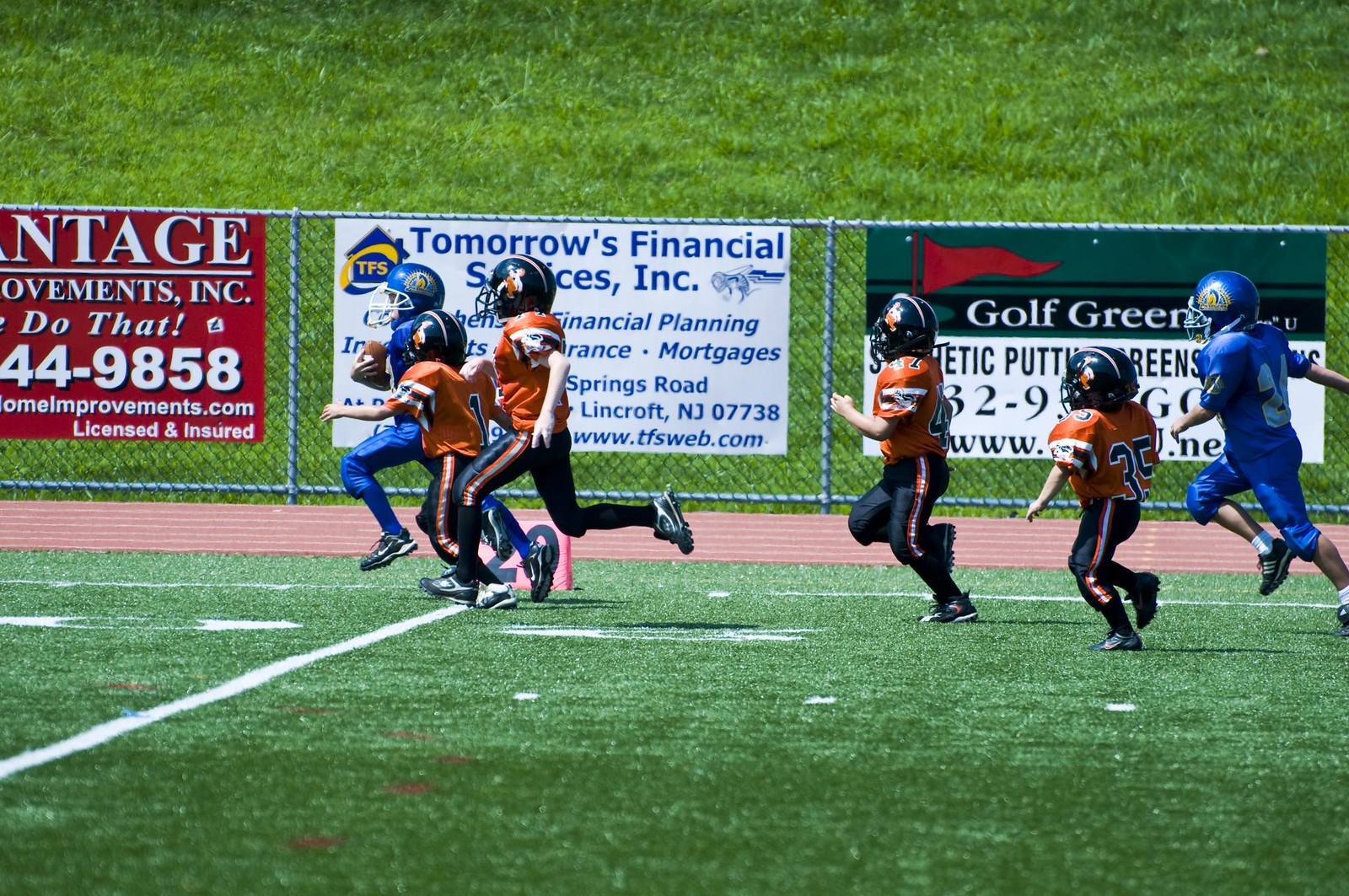This photograph captures a lively American football game featuring young children on a vibrant green sports field. In the image, six players are seen running towards the left. The lead player, dressed in a blue uniform, clutches the football tightly. The remaining players chase after him, all donned in orange and black uniforms, with each player wearing a helmet. A metallic fence adorned with various sponsor posters and advertisements—one red and partially cut-off, another white with "Tomorrow's Finance Financial Services Inc," and a third promoting "Golf Green"—borders the field. The lush green grass extends beyond the fence, punctuated with some brown patches in the lower left corner, enhancing the sporty and energetic atmosphere of this children's game.